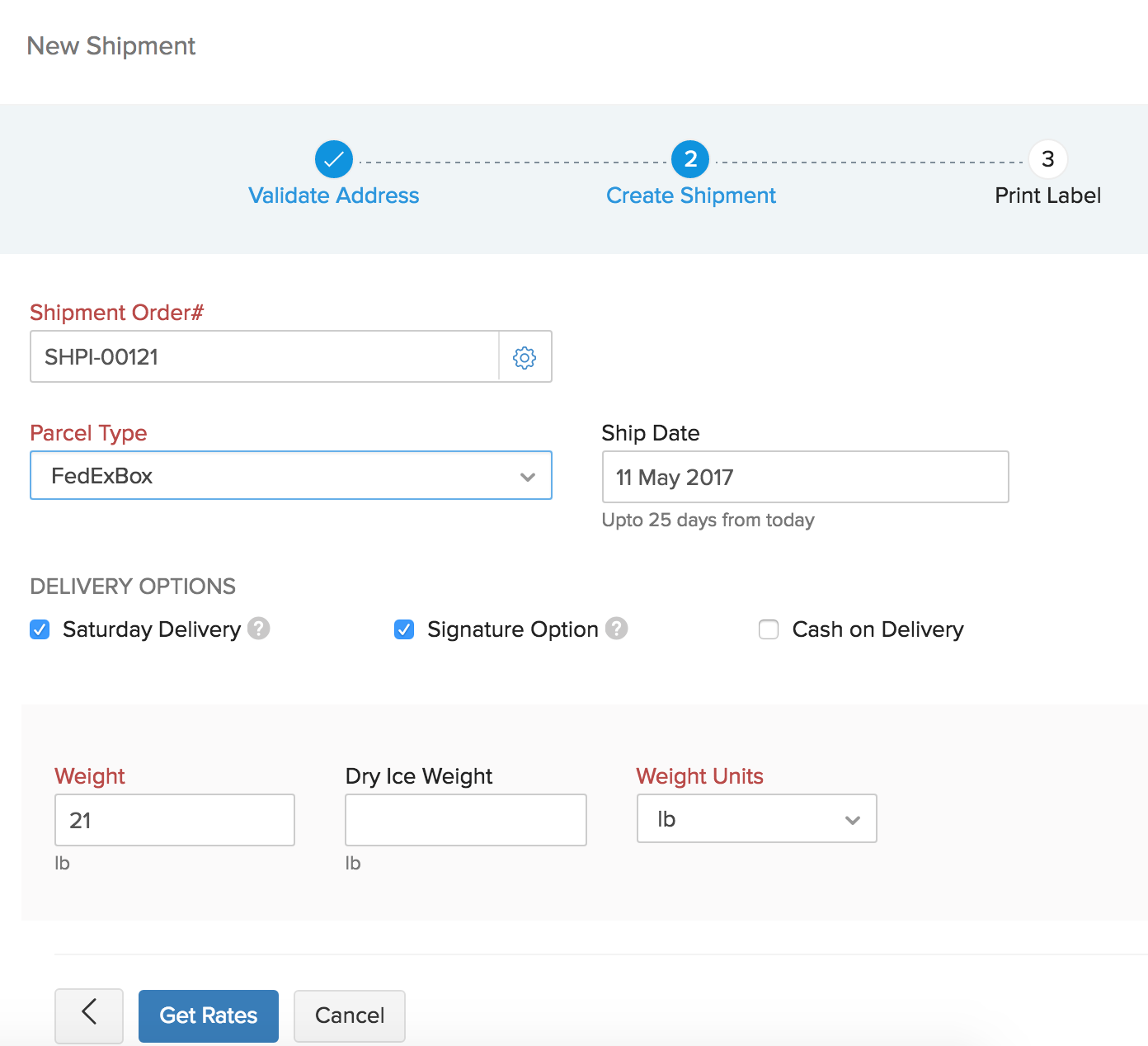The image depicts an online shipment creation process, broken down into three sequential steps, with the current focus on step 2 of 3. The steps are clearly outlined as follows: 

1. *Validate Address* - marked complete with a green checkmark.
2. *Create Shipment* - the current active step.
3. *Print Label*.

Below the steps, there's a shipment order form. The order number is specified as SHPI-00121, with a gearbox icon adjacent to it for modifying the order number if needed. The "Parcel Type" field has been set to "FedEx Box" but is changeable via a dropdown menu. Next, the "Ship Date" is displayed as May 11, 2017, indicating it's set to be shipped within 25 days from today.

Under "Delivery Options," "Saturday Delivery with Signature" is selected. There's also a question mark icon next to it for additional information. The "Cash on Delivery" option is visible but not selected.

Beneath the delivery options is a light gray "Weight Details" box, which includes fields for "Weight," "Dry Ice Weight," and "Weight Units." The current weight is listed as 21 pounds, with no value for dry ice. The units are set to pounds, but this can be adjusted. 

At the bottom of the form, there are three buttons: "Get Rates" in blue with white text, a "Cancel" button to the right, and a "Back" button to the left.